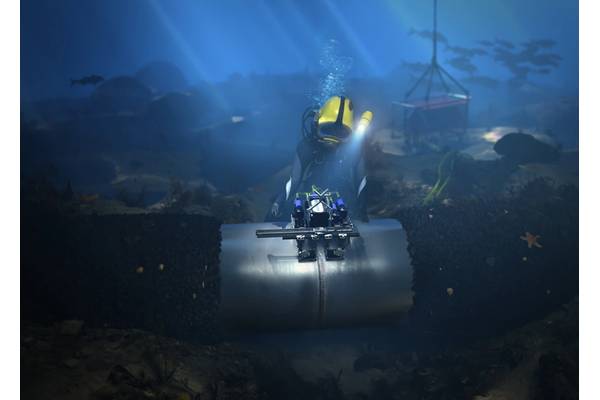This image depicts an underwater scene featuring a scuba diver engaged in what appears to be inspection or repair work on a large metallic structure lying on the ocean floor. The diver, clad in a grey scuba suit and distinctive yellow helmet, emits bubbles from their breathing apparatus. They are illuminated by a work light mounted over their left shoulder, which casts focused rays onto the machinery in front of them. This contraption includes a wide metallic tube adorned with blue cylinders and a suspicious-looking device that resembles an explosive.

In the background, a crane's rope extends downward, maneuvering a box lifted off the seabed, suspended by four chains. The underwater environment is slightly beige and sparse, with pockets of marine foliage and a starfish clinging to a piece of netting near the metallic structure. Additionally, the scene includes blurred schools of fish swimming and faint sun rays filtering from the surface, adding to the picture's rich detail. A cage can be seen in the distance, presumably used for the diver's ascent and descent.